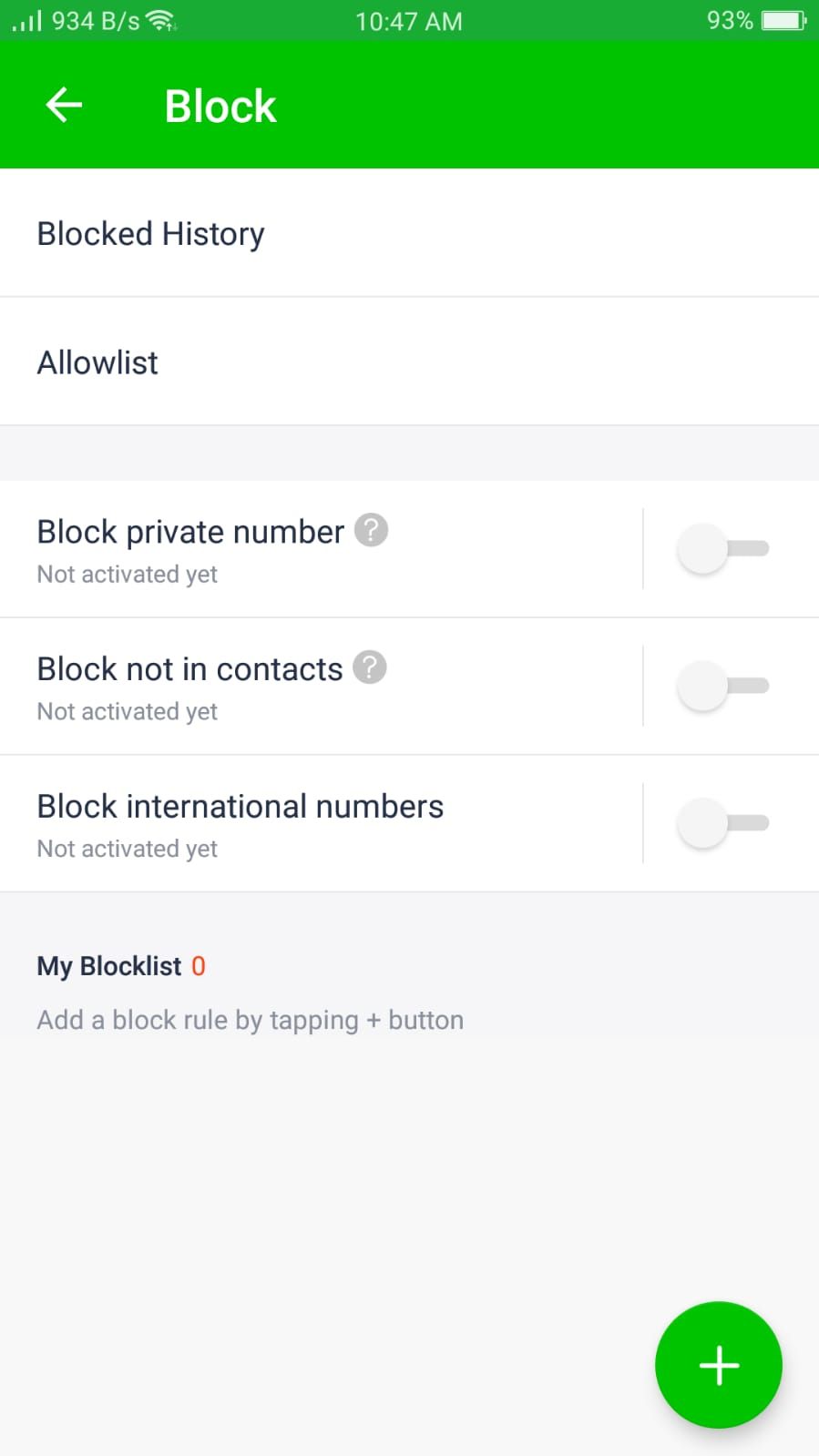The image is a screenshot of a block settings page from a mobile device. At the top, there is a bright green header displaying the title "Block Settings," with a left-facing arrow in the top left corner for navigating back to the previous page. Below the header, there is a list of settings.

The first two settings are "Blocked History" and "Allow List," each separated by a small space. Following these are three additional settings:
1. "Block Private Numbers" - Accompanied by a small question mark icon for more information. Beneath the title, there is lighter-colored text stating "Not activated yet."
2. "Block Calls Not in Contacts" - Also featuring a question mark icon with a sub-description in lighter text reading "Not activated yet."
3. "Block International Numbers" - This setting does not have a question mark icon but includes a sub-description that says "Not activated yet."

All three of these settings have toggles on the right side, which are grayed out and switched off.

Towards the bottom of the list, in bold text, is "My Block List" accompanied by a red "0." Beneath this, a description reads, "Add a block rule by tapping the plus button."

The final item on the page, located at the bottom right-hand side, is a large green circular button with a white plus icon in the center, used for adding new block rules.